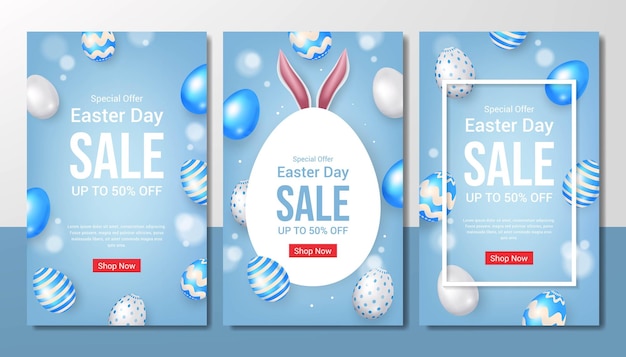The image is a screenshot of a display ad, possibly featured on a website, promoting an Easter sale. The advertisement consists of three vertical rectangles arranged side by side, each with a beautiful sky blue background color. 

Surrounding the rectangles, there is a dual-colored border – light lavender on the top and a slightly darker shade of blue at the bottom. The center rectangle prominently features a white egg shape with pink rabbit ears on top. Written in blue font on the egg is the text "Easter Day Sale, up to 50% off." Below the text is a red rectangular button with the words "Shop Now" in white.

The background within this central rectangle is adorned with tiny, decorated Easter eggs, adding a festive touch. The rectangles on either side of the central image share the same sky blue background and egg decoration but do not feature the white egg icon. Instead, they simply display the text "Easter Day" with the word "Sale" in a large white font. The overall design effectively evokes the spirit of Easter with its vibrant colors and playful imagery.